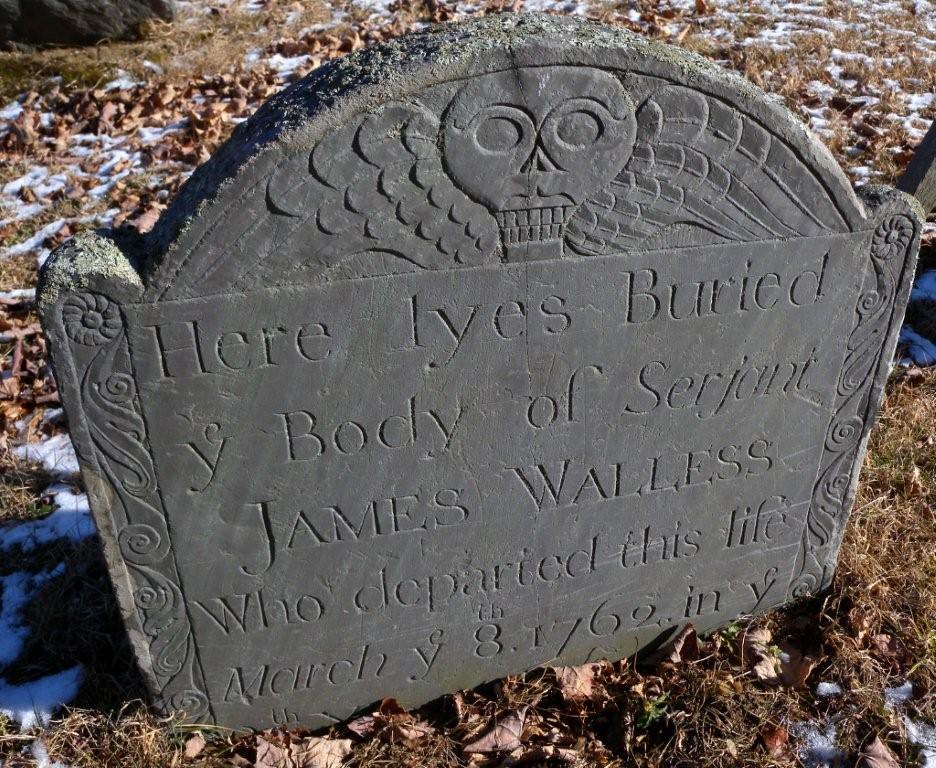The image captures a weathered, dark gray tombstone with a rounded top, positioned in a graveyard amidst a cold landscape. The ground is littered with dry, crumpled leaves and sparse patches of brown grass, interspersed with spotty areas of snow, indicating it was taken in early spring or possibly late winter. Natural daylight is evident, as the tombstone casts shadows on the snowy and grassy ground surrounding it. The top of the headstone displays a carved winged skull, adding an eerie, aged aura to the scene. The inscription reads, "Here lies buried the body of Sergeant James Wallace, who departed this life March 8, 1769," marking it as a relic from the 18th century. The tombstone, showing signs of significant age and wear, evokes a sense of somber history and timelessness.